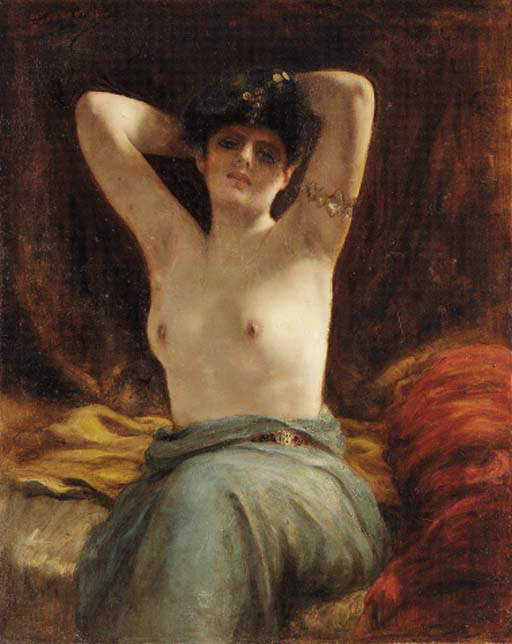In this old-fashioned painting, an Eastern European woman with dark hair styled up holds her hands behind her head, exposing her upper body, which is uncovered above the waist. She is sitting on a bed adorned with red, orange, and yellow bedding, which contrasts with her greenish-blue dress that has fallen to her waist, resembling the color of sea foam. The woman's gaze is directed at the camera, exuding a confident demeanor. Her accessories include a gold bracelet worn high on her arm. The backdrop is a dark, mottled brown, further highlighting the richness of her red lips, dark eyes, and the slight underarm hair visible as she lifts her arms.